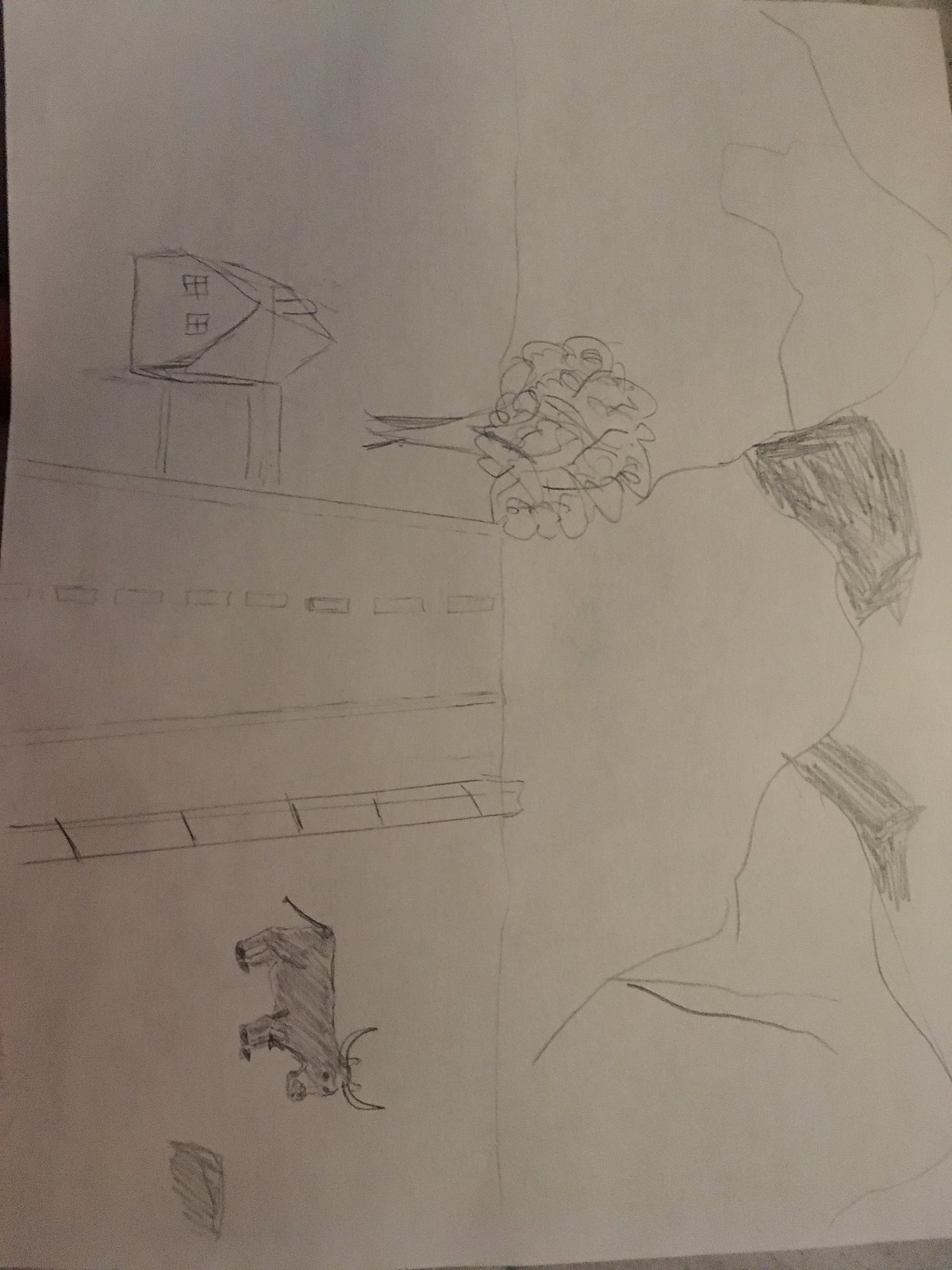This detailed pencil sketch is drawn on a white piece of paper and is currently rotated 90 degrees sideways. The scene is presented from an angled perspective, making the horizontal orientation appear vertical. Dominating the right side of the image is a large cow, distinguished by its prominent horns and black tail, standing next to a rock in what seems to be a pasture enclosed by a fence. On the left, there is a small house that closely resembles a barn, featuring two windows at the top, a chimney, and a slanted roof. A road with dotted lines runs between the pasture and the house, curving around in the sketch. Behind the house, a tree with a uniform, straight trunk and a dense, bushy canopy is visible. In the background, rolling hills or mountains complete the picturesque setting. The bottom right corner of the image reveals the surface on which the paper is placed, further emphasizing the sideways orientation of the drawing.